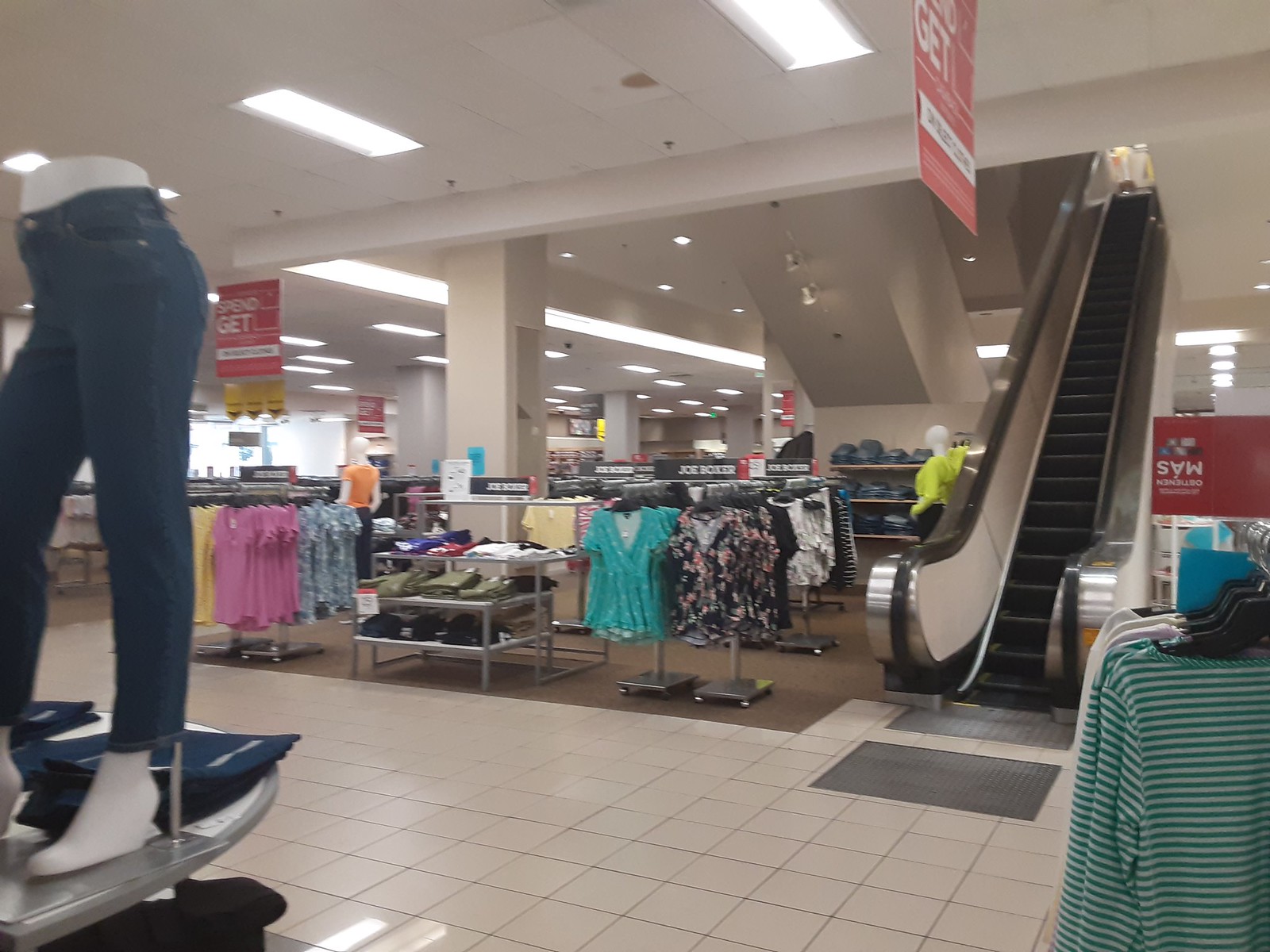This image depicts the interior of a department store, likely Macy's, with several distinctive features that make it a detailed scene. The store has a typical layout with ceramic tile floors in the high traffic areas and carpeting around the clothing racks. A silver escalator can be seen descending from the second floor, indicating that the store has multiple levels. To the left of the image, a mannequin from the waist down showcases some jeans and white shoes, while to the right, green and white striped polo shirts hang on black hangers. The brightly lit ceiling, adorned with fluorescent lights, casts light over numerous clothing displays, which include racks of blue shirts, black and pink floral shirts, and other assorted apparel neatly folded on silver display tables. There are also several red and white signs spread throughout the store, and additional mannequins are posed to model the latest styles, emphasizing the wide selection of women's clothing available in this section.